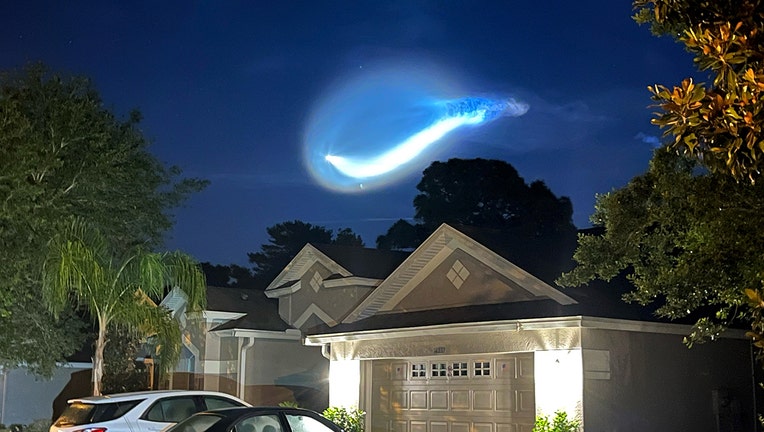The image depicts a nighttime scene in a suburban neighborhood, with the primary focus on a bright white flare or trail of light streaking across a dark blue sky, suggestive of a rocket or some other luminous entity. Framed by this celestial phenomenon, the foreground showcases three suburban beige houses with black-shingled roofs, underlined by white trim and garage doors. Two vehicles, one white SUV and one black car, are parked in the driveways. The environment is complemented by an assortment of trees, including palms and large ficus trees, adding depth and framing to the composition. While the image has the appearance of a digital design or painting, the meticulous details and striking contrast between the serene neighborhood and the mystical sky make it captivating.